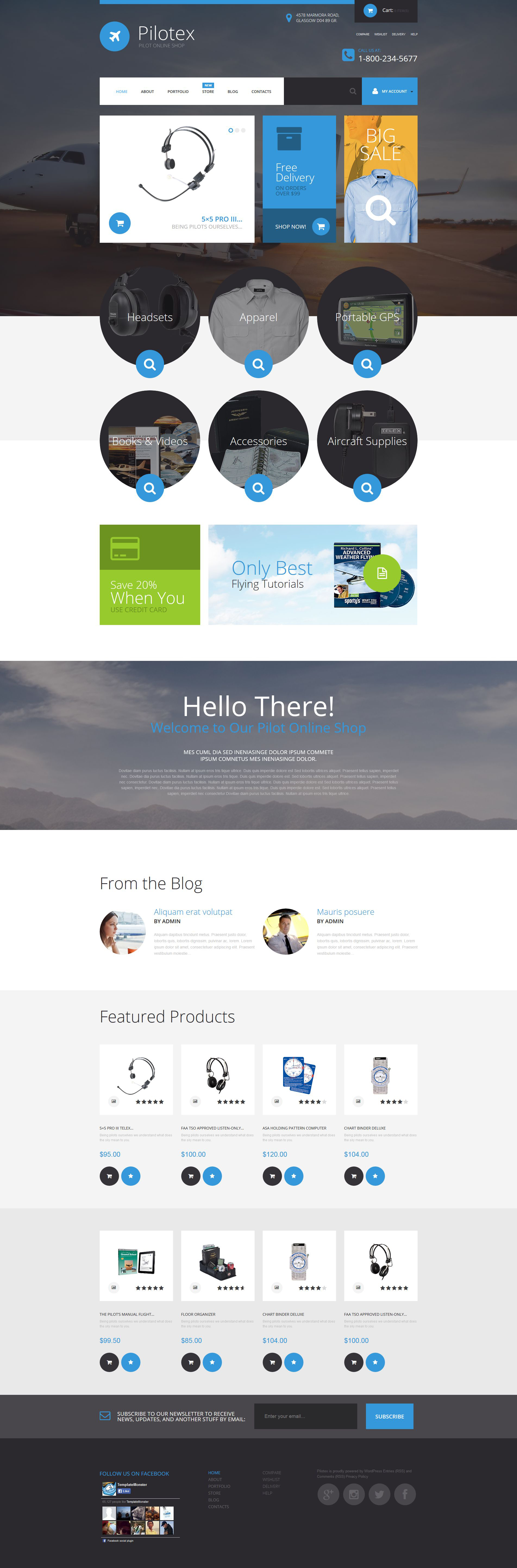**Caption:**
Screenshot of the Pilotex website interface, showcasing various navigation elements and featured products. The navigation bar at the top includes "Home, About, Portfolio, Store, Blog, Contacts," next to a search bar and "My Account." The site is identified by a blue circle featuring a white airplane icon next to the name 'Pilotex'. Contact information and helpful links such as "Cart, Compare, Wishlist, Delivery, Help, Call us at 1-800-234-5677" are also present. The background features an image of an airplane, enhancing the aviation theme.

Promotional banners highlight products like the 5x5 Pro 3 headset, with the phrase "being Pilots Ourselves," and offer free delivery on orders over $99 with "Big Sale" announcements. Categories like "Headsets, Apparel, Portable GPS, Books and Videos, Accessories, Aircraft Supplies" are listed, along with a savings note: "Save 20% when you use credit card". 

A welcome message reads, "Hello there, welcome to our pilot online shop," followed by placeholder Latin text over a background image of a mountain range under a blue sky. 

The "From the Blog" section has more placeholder text, while "Featured Products" showcases items like the "5x5 Pro 3 Telex FAA TSO Approved Listen Only - $100," "ASA Holding Pattern Computer - $120," "Chartbinder Deluxe - $104," "The Pilot's Manual Flight - $99.50," and "Floor Organizer - $85." 

At the bottom, users are encouraged to "Subscribe to our newsletter to receive news, updates, and other stuff by email," with a subscription box for entering email addresses. Social media engagement is prompted with a "Follow us on Facebook" call-to-action.